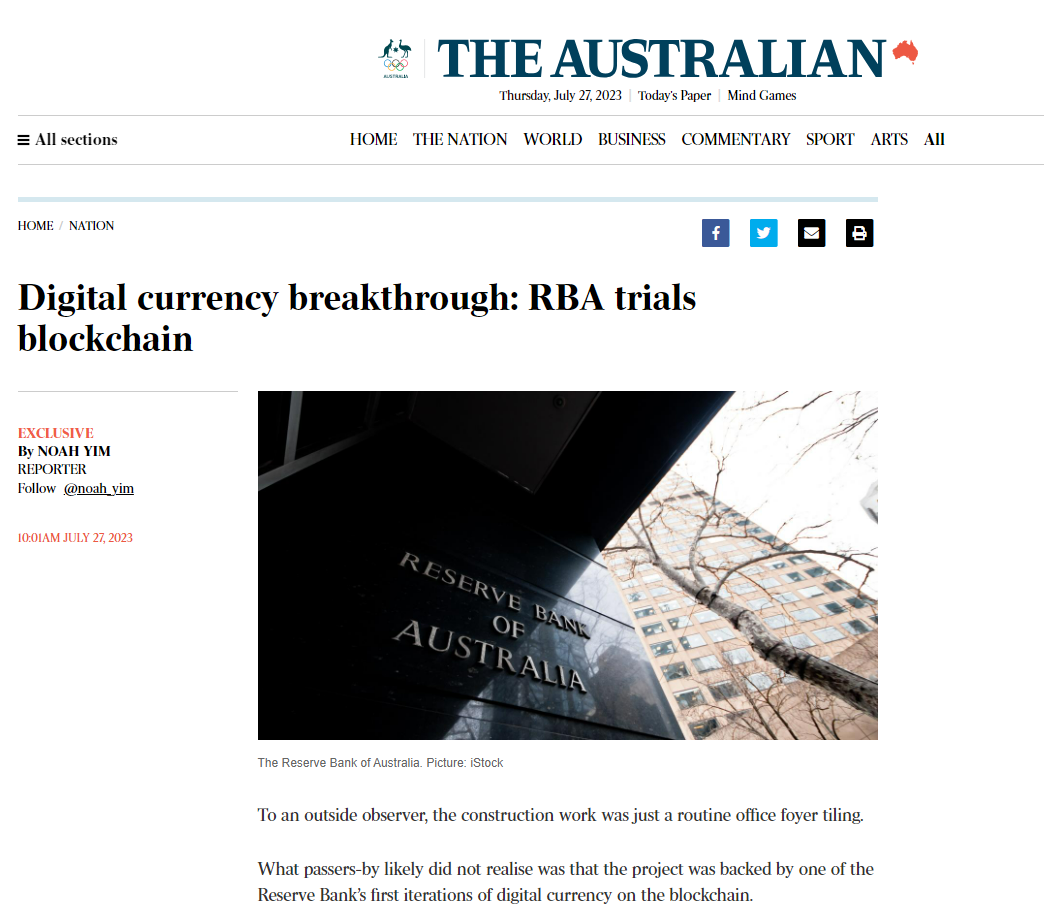The image displays the homepage of "The Australian" website. To the left, there is an Olympic-themed logo, and to the right of "The Australian" title, a red silhouette representing the continent of Australia is prominently featured. The header indicates the date, Thursday, July 27th, 2023, along with the headline "Mind Games" and navigation options for various sections: Home, Nation, World, Business, Commentary, Sport, Arts, and All.

Highlighted in the section "Home/Nation" is an article titled "Digital Currency Breakthrough, RBA Trials Blockchain," marking it as an exclusive piece authored by reporter Noah Yim. The author’s Twitter handle, @Noah_Yim, is also provided along with the publication time and date: 10:01 AM, July 27th, 2023. Accompanying the article is a stock photo from iStock featuring the Reserve Bank of Australia. The initial lines of the article suggest that what appeared to be routine office construction work to passersby was, in fact, related to the Reserve Bank's initial implementation of a digital currency using blockchain technology.

Additionally, the interface includes typical sharing options for social media platforms such as Twitter and Facebook, and options to print the article.